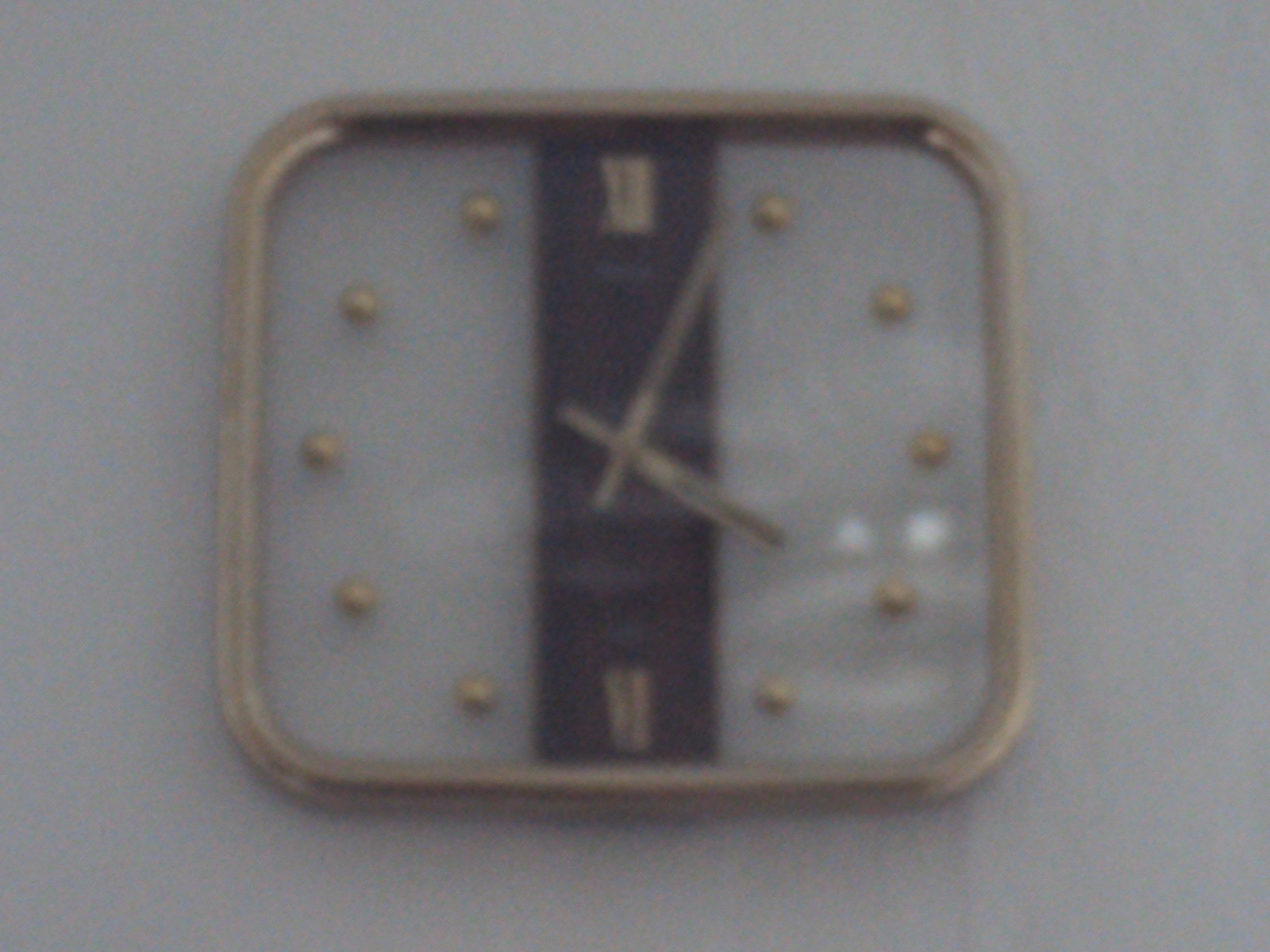The low-resolution, slightly out-of-focus image features a square-shaped wall-mounted clock. The clock has a golden or chrome metallic frame with rounded edges, positioned centrally against a light gray or white background. The clock face itself presents a minimalist design with a vertical black strip running down the center, upon which the golden metallic hands are affixed. At the 12 and 6 positions, there are small Roman numerals in gold, while the other hours are indicated by golden dots or buttons spread evenly around the white face. The time displayed reads approximately 4:03 or 4:05. The glass face of the clock reflects ambient light, adding to the subtle blurriness of the image.